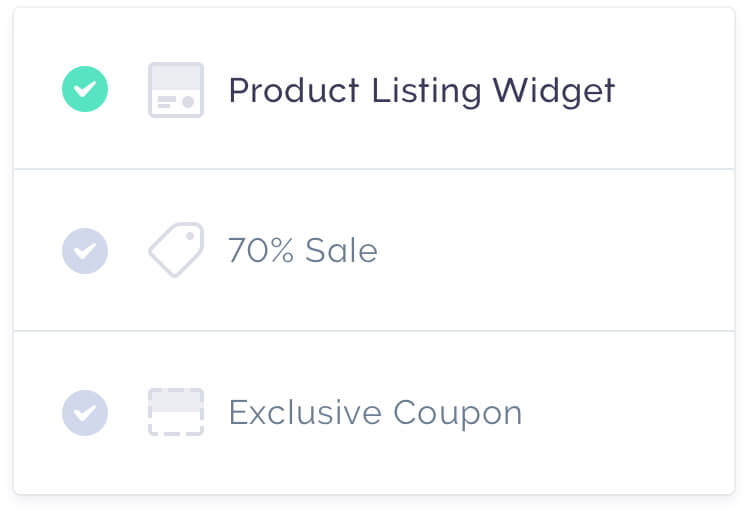The image features a clean white background with three prominent rectangular sections, each outlined in light blue. 

1. The first section displays a green circle with a white check mark inside, accompanied by a small blue square. Beneath this image, the text reads, "Product Listing Widget."
2. The second section shows a blue square with a white check mark, next to a small price tag icon. The text below this section states, "70% Sale."
3. The third section contains a blue circle with a white check mark, accompanied by a blue dotted box that is half blue and half white inside. The text here reads, "Exclusive Coupon."

Each section's icon effectively represents its respective feature, making the overall image a concise visual summary of the product offerings.